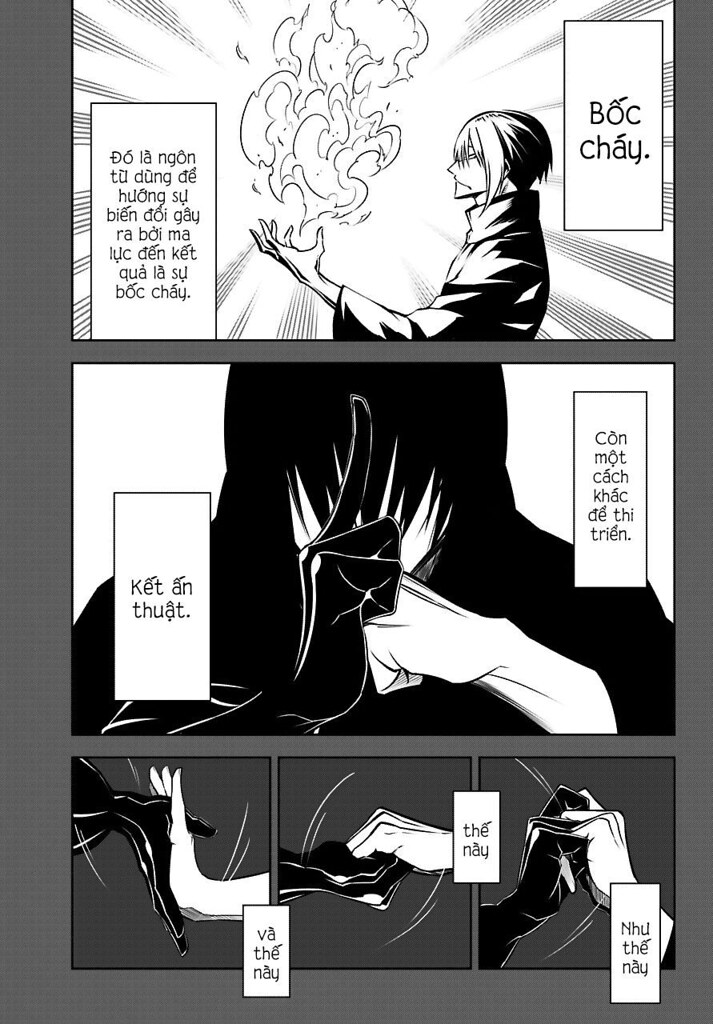The image is a manga-style comic strip consisting of three vertically stacked panels, all rendered in black and white. The comic seems to be in a foreign language, featuring text in rectangular boxes scattered throughout.

**Top Panel:** A female character, shown in a side profile, appears visibly annoyed or angry. She holds her hand out in front of her, with fingers slightly clenched, releasing what looks like smoke or fire. Her mouth is downturned, emphasizing her emotional state. There is text in rectangular boxes to both the left and right of her figure.

**Middle Panel:** This close-up frame highlights a person in silhouette or dressed entirely in black, including a dark covering over their face. The main focus is on their hands: one is black and holding up an index finger, while the other, a white hand, is balled into a fist and is pressed into the palm of the black hand. Several rectangular text boxes are visible on either side of the image.

**Bottom Panel:** This strip is divided into three separate images, each intensifying the interaction between a black hand and a white hand. In the first image, the black hand faces down, meeting the white palm facing up. The second image shows the hands interlocked, fingers intertwined. In the final image of this panel, both hands form fists, lightly touching each other, with some fingers forming a slight steeple shape. Text boxes, presumably explaining these interactions, accompany each sub-panel.

The comic is bordered in gray along the left, bottom, and right sides, adding a framed effect to the detailed monochrome art.